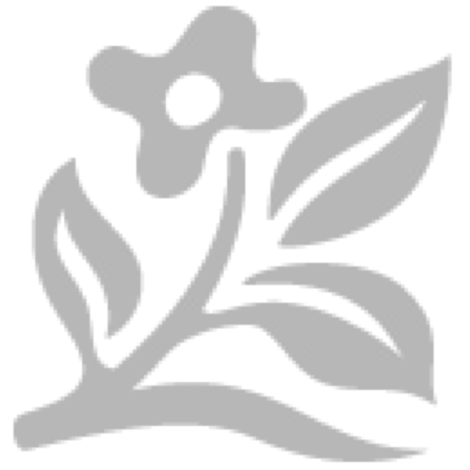This captivating high-resolution photograph showcases vibrant magenta, bell-shaped blossoms basking in direct sunlight. In the foreground, three distinct stems are depicted with striking sharpness and clarity. Each stem supports clusters of around 10-12 tiny flowers, with petals partially opened in various stages of bloom. The blossoms flaunt yellow-green stamen with delicate orange filaments at their centers. The flowers, devoid of foliage at their tops, reflect hues of greenish-yellow and reddish on the stems. Background elements are artistically blurred, highlighting more delicate blossoms and verdant leaves. This image, seemingly taken in daylight, exudes a garden-like ambiance filled with these intricate clusters flaunting their delicate beauty.